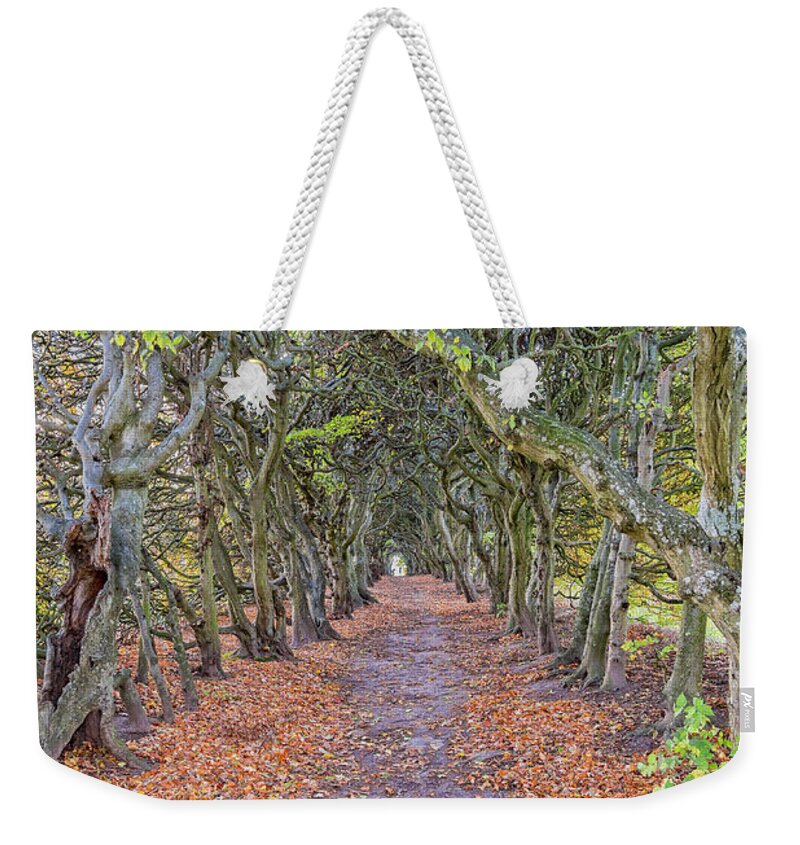This image showcases a rectangular tote bag featuring a detailed, printed illustration of a serene forest scene. The forest is depicted with a pathway running through the middle, surrounded by scattered, brown, muddy-looking ground and an array of fallen leaves in hues of orange, dark red, and yellow. The trees lining the pathway have mostly barren branches with a few scattered green leaves, and some are tinged with green algae. The bag itself is equipped with white, fabric cord handles, adding a touch of practicality to its design. The natural and serene setting is captured with a high level of realism, presenting a harmonious blend of nature and everyday utility.